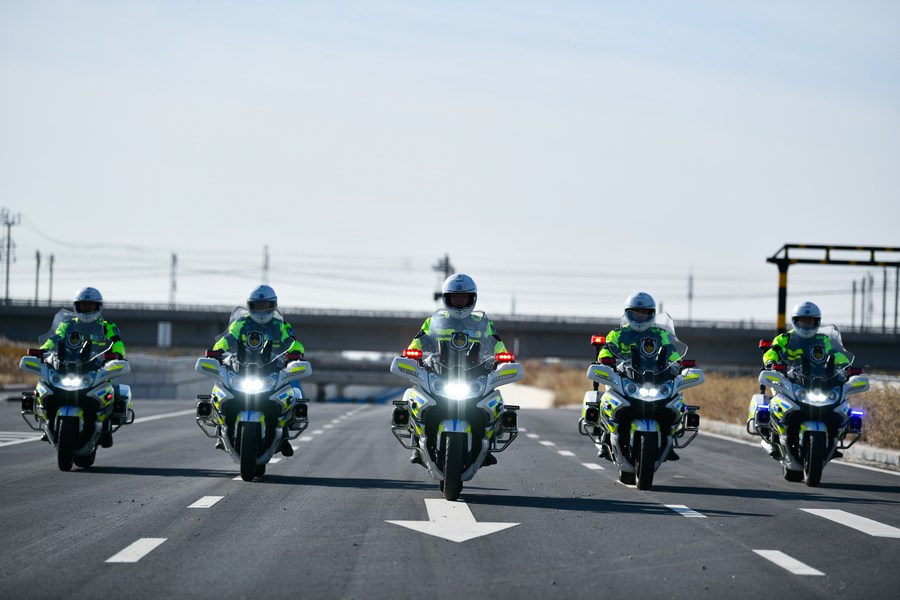In this vibrant afternoon highway scene, five motorcyclists, evenly spaced in a nearly perfect line, ride towards the viewer on an expansive asphalt freeway. Each rider is clad in identical neon green safety vests over puffy jumpsuits, paired with white helmets featuring bug shields. Their motorcycles, or possibly scooters, mirror each other exactly, indicating uniformity and perhaps a club association. The perspective centers on one rider, flanked symmetrically by two on either side, all highlighted by a forward-facing arrow on the road beneath. This scene unfolds under a flat, light sky with blurred details, featuring two freeway overpasses in the background and telephone lines crossing above. Construction activity is faintly visible to the right, adding a touch of industrial atmosphere to this dynamic, safety-conscious convoy.